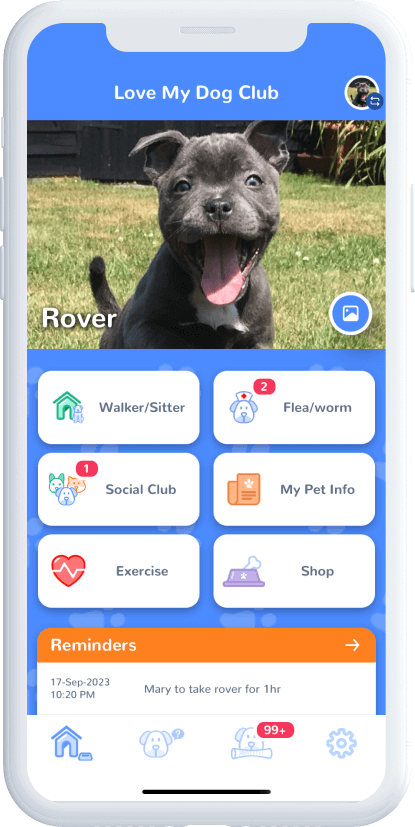The image features a mobile phone with a sleek white exterior. The top part of the phone showcases the speaker. On the left side, there are three buttons: the volume up button, the volume down button, and the power button. Additionally, there is another button situated on the right side.

Displayed on the phone’s screen is an app with a blue background and a prominent title at the top center that reads "Love My Dog Club" in white, with each word capitalized. Below the title, there is a grassy area featuring a black puppy named Rover, as indicated by the text "Rover" at the bottom left corner within a black-bordered and shadowed rectangle. 

In the bottom right corner of the screen, a blue circle with a white border contains an image icon, suggesting users can click it to add an image. Below the main image area, six rectangular menu options with white backgrounds and rounded edges are visible:
1. Walker/Sitter
2. Social Club
3. Exercise
4. Flea/Worm
5. My Pet Info
6. Shop

An orange header labeled "Reminders" is found at the bottom of the screen, written in white with a white arrow beside it. Below this header, the reminder text is displayed in gray: "17-SEP-2023 10:20 PM Mary to take Rover for one HR."

At the very bottom of the screen, there is a menu bar containing several icons:
- A dark blue 3D doghouse on the left, indicating it is selected.
- A light blue dog face.
- Another light blue dog face with a bone, accompanied by a red oval in the top right corner displaying the number 99.
- A gear icon on the far right, indicating settings or configurations.

The detailed layout of the app provides a user-friendly interface for dog owners, featuring various options to manage and care for their pets.